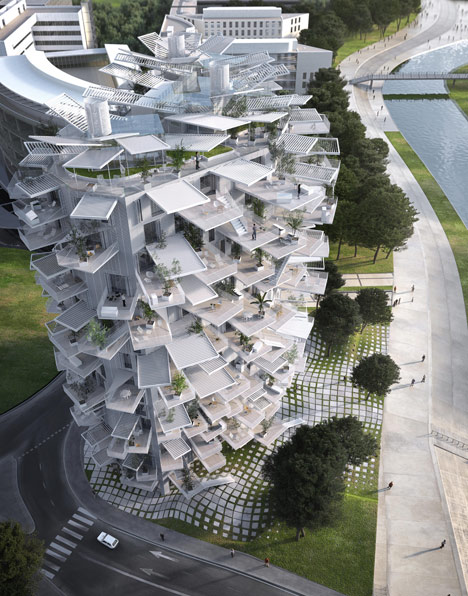The image features an intricate 3D rendering of a futuristic, concept high-rise building. The building, resembling a pine cone, stands upright with a distinctive spiral shape, composed of numerous levels that could make it either a pioneering apartment complex or a monumental structure. Each of the many floors extends outward in the form of thin, rectangular white balconies laden with potted plants, including palm trees and various green shrubs, adding a touch of nature to the architectural design. The balconies appear to be very slim, almost paper-like in their delicacy. Surrounding the base of the building is a large blacktop road that spirals around it, and a sizable gray cement walkway flanks the structure. Adjacent to the walkway, there is a bridge spanning a river, enhancing the scene with dynamic elements of both natural and urban landscapes. Trees and bushes line the walkway, providing a lush backdrop against the innovative building. The top of the image features a curved element that may function as a driveway, contributing to the overall pine cone-like appearance. The rendering captures the essence of blending nature with avant-garde architecture.